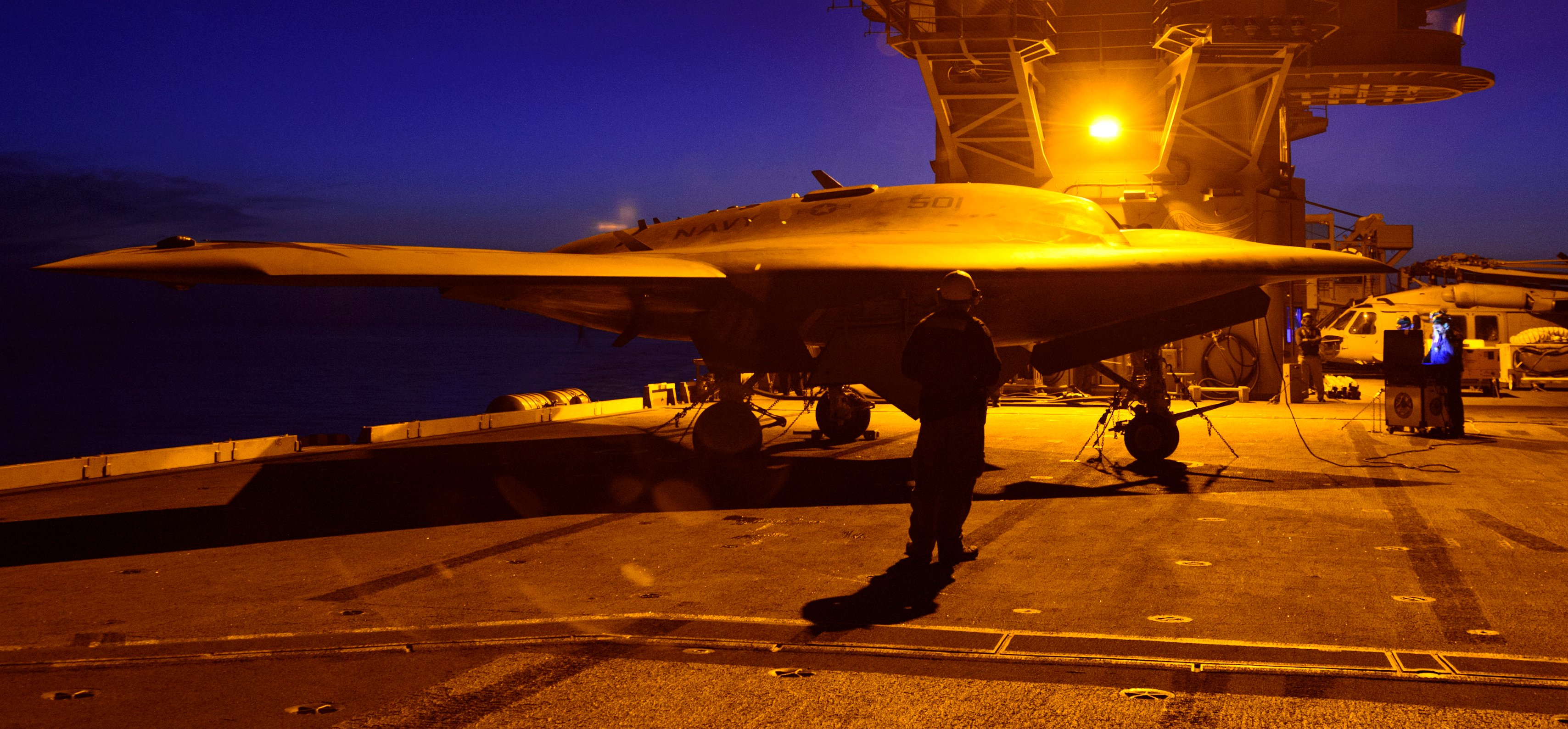In this nighttime image, we see a detailed scene on an aircraft carrier's deck, shrouded in a dark blue sky. Dominating the foreground is a Navy fighter jet, marked with the number '501' and the Navy insignia. The jet, facing towards the right, displays its left wing clearly while something stands underneath it, possibly a support stand. Positioned at the center of the image is a man in a helmet and black work suit, his back to us as he faces the jet, indicating his role in pre-flight or post-flight operations. To the right, three other personnel, clothed in blue airsuits, are gathered around an open box with light emanating from inside. The carrier's deck features a control tower in the background, emitting a bright light that casts shadows around. Helicopters and additional aircraft, appearing as silhouettes, dot the background amidst various support vehicles and equipment trailers, adding depth and context to the vibrant yet shadowy scene.